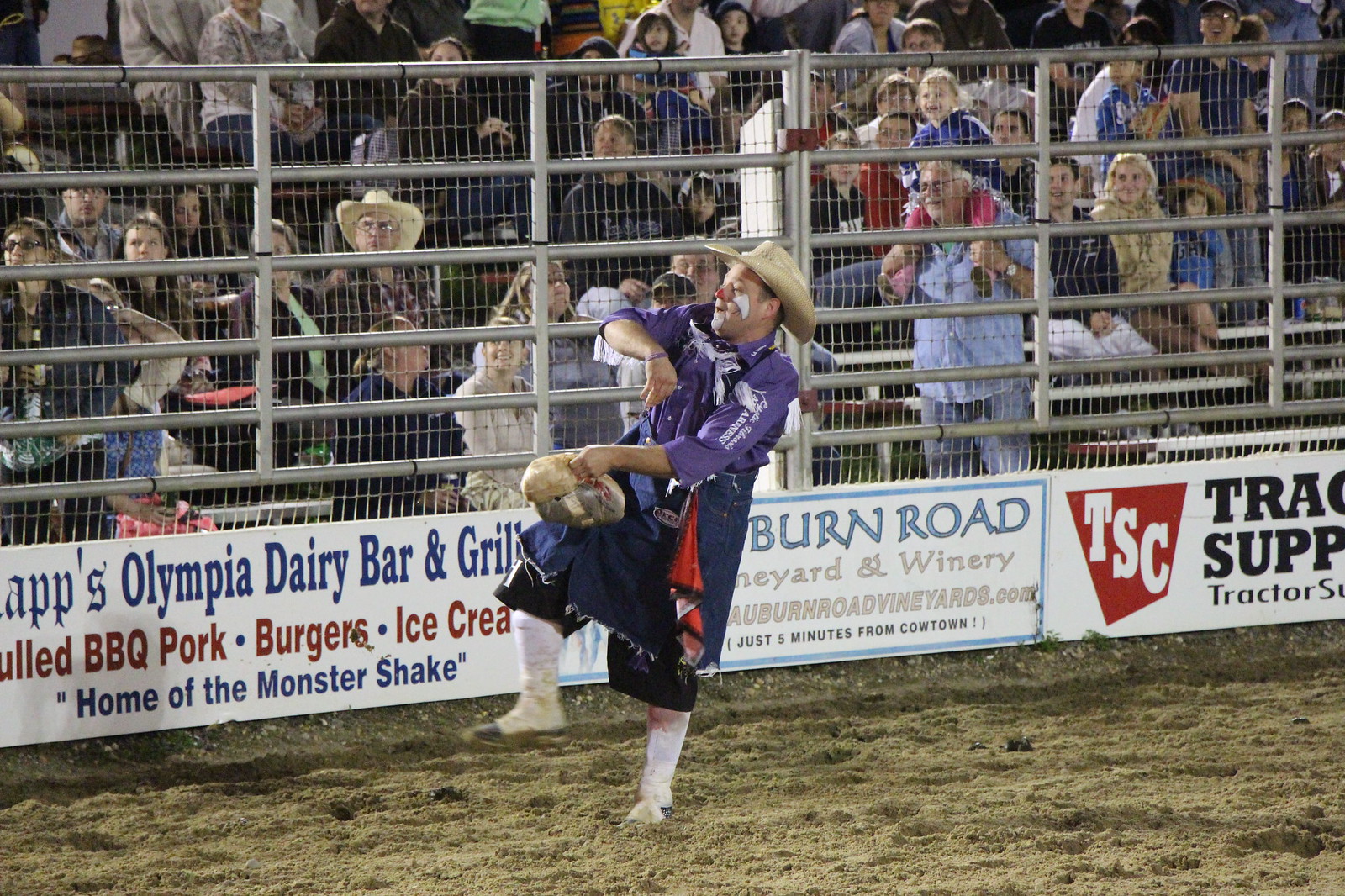This is a detailed photograph capturing the vibrant atmosphere of a rodeo event. In the foreground, a rodeo clown, dressed in a purple shirt, black shorts, and a cowboy hat, stands strikingly on one leg with his right leg lifted in the air, facing to the side. His face is adorned with clown makeup, featuring a painted red nose and white cheeks, and he appears to be holding a mask in his hand. The clown is also wearing white long socks or strappings that resemble boots.

The ground he stands on is a typical light brown, dirt turf characteristic of rodeo arenas. Surrounding the arena is a sturdy gate-like barrier and netting, designed to protect the audience, who are visible in the packed grandstands behind the clown. The spectators' faces are turned towards the action, indicating an engaging spectacle that is not captured within the frame.

Above the gate, a series of colorful sponsor banners can be seen, advertising local businesses such as Olympia Dairy Bar and Grill, Pulled Pork, Burgers, Ice Cream, Homo the Monster Shake, Burn Road Vineyard and Winery, and TSC Tractor Supply Company. These ads highlight the community spirit and commercial support for the event. Overall, this image perfectly encapsulates the lively and communal essence of a rodeo.